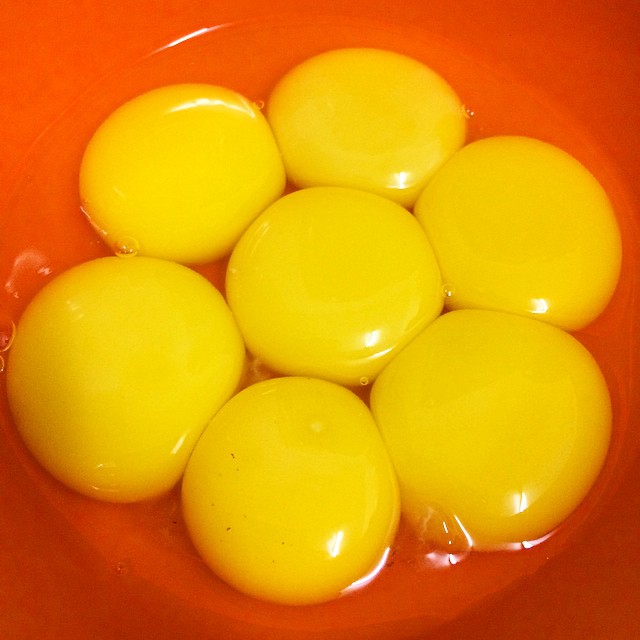This photograph captures a detailed close-up of seven bright yellow egg yolks arranged in a distinctive pattern within a red, possibly reddish-orange bowl. The egg yolks, which are raw and unbroken, are clustered closely together, with one yolk positioned in the center and the remaining six forming a ring around it. These yolks float in a clear egg white, through which small bubbles are visible, adding to the texture of the image. The high level of lighting enhances the shiny, reflective surfaces of both the yolks and the bowl, highlighting intricate details such as reflections of light on the yolks. Overall, the egg yolks dominate the frame, creating a visually striking composition against the vibrant red of the bowl.